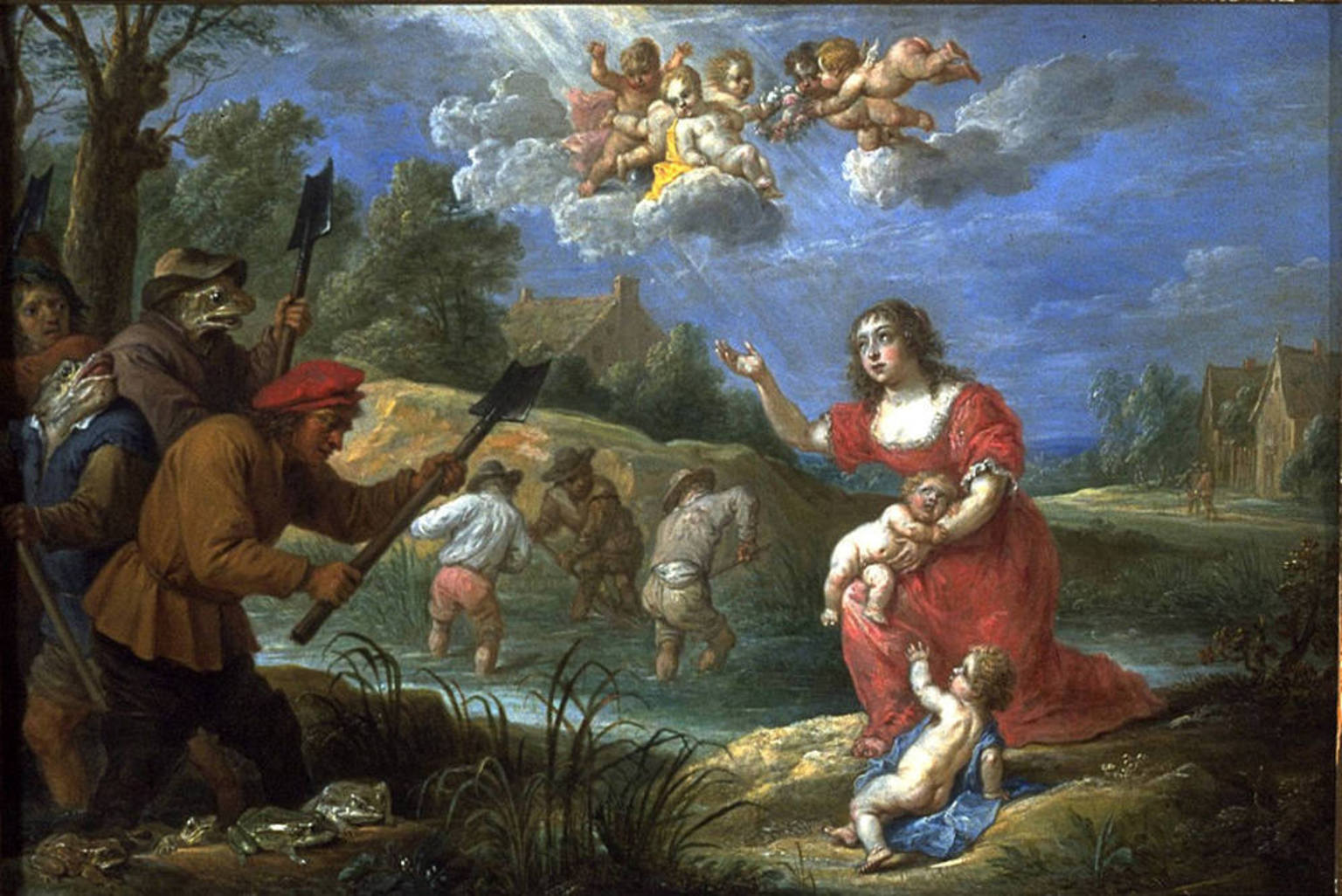In this intriguing oil painting, the scene is set under dark blue skies filled with clusters of clouds. Among the clouds, cherub-like babies reminiscent of cupids appear to be engaged in a playful tug-of-war with a floral garland. The right and left sides of the image are populated with quaint houses, while a small village is visible in the background, providing a serene backdrop to the intense foreground activity.

Central to the composition is a woman dressed in a striking red dress, seated by a lake or swamp. She holds a naked baby on her lap, shielded by a blue blanket, and another naked baby rests on the ground beside her. The woman, seemingly illuminated by rays of light streaming through the clouds above, looks skyward with one hand extended, adding a divine or contemplative element to the scene.

On the left-hand side, a group of men, possibly farmers, are gathered along a riverbank. They are engaged in some laborious activity, possibly digging or shoveling, with long-handled tools. Interestingly, two of the men appear to have frog heads, and there are several toads scattered at their feet. Unlike the illuminated woman, these men remain shaded, untouched by the heavenly light.

Overall, this painting blends celestial and earthy elements, contrasting the serene and the laborious, the divine and the mundane, into a richly detailed and complex tableau.